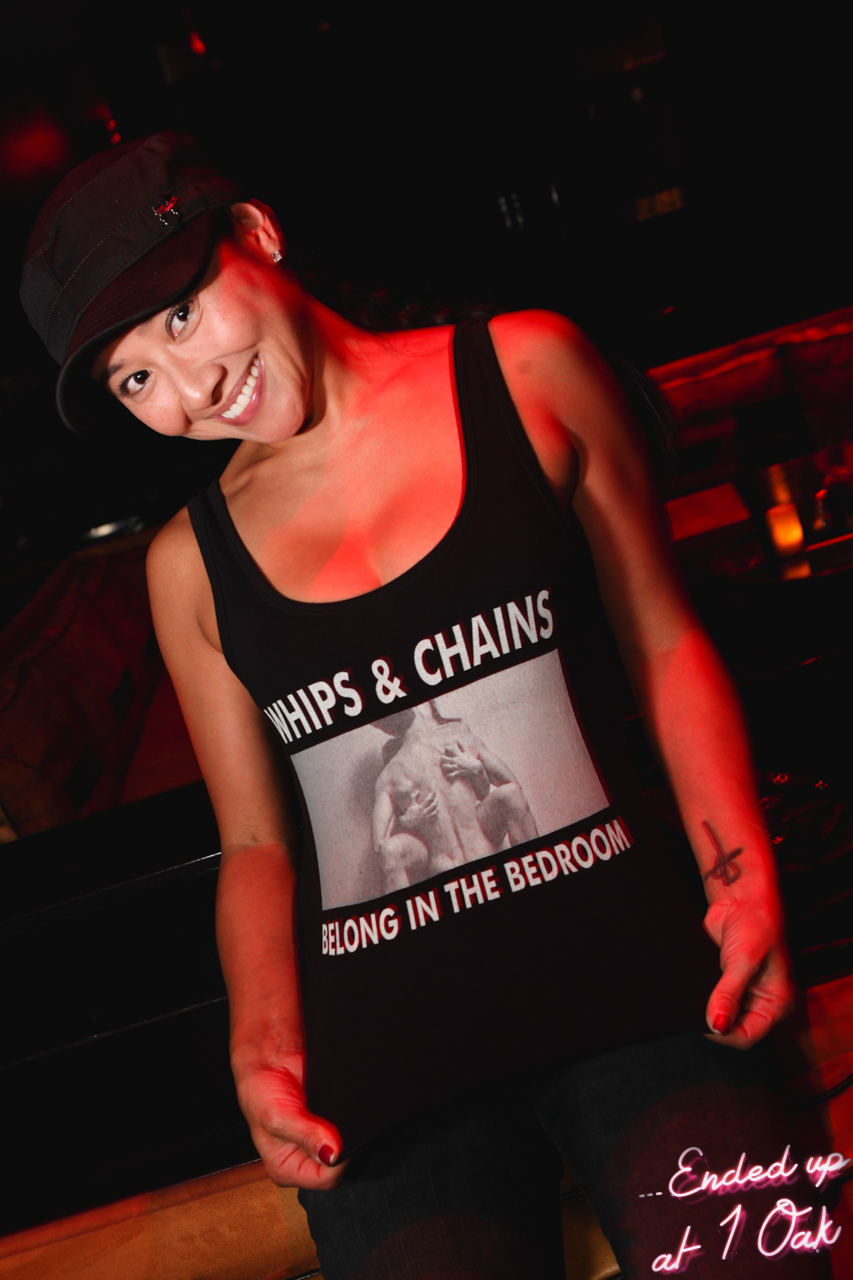The photograph captures a young woman posing confidently in a very dark nightclub. She stands with her head cocked to the right, a broad smile showing her teeth. She is sporting a black baseball cap adorned with a shiny metallic pin on the front. Her ears glint with gem-studded earrings. The woman is dressed in a sleeveless black graphic tank top, which is low-cut. In bold white text, her top reads, "Whips and chains belong in the bedroom," surrounding a graphic picture of two naked individuals holding each other. She pairs this with black tights and displays a tattoo of an inverted cross on her left wrist. In the dim surroundings, characterized by multiple couches, low tables with lit candles, and some red ambient lighting, the club's mysterious ambiance is palpable. The bottom right of the photo features pink font text, adding an extra touch to this captivating scene. This setting, identified as One Oak nightclub, suggests a potential special event focused on adult themes.